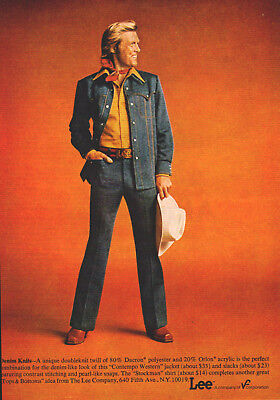The image is an old advertisement for Lee Jeans, likely from the 1970s, characterized by its distinctive vintage style. A man with medium-length, sandy blonde hair stands against a burnt orange background. He wears a matching denim jacket and pants with slightly flared bottoms, a mustard yellow collared shirt underneath, and a red bandana tied around his neck. The man sports brown leather shoes and a noticeable large belt with a prominent metal buckle. He's holding a white cowboy hat in his right hand, with his left hand tucked into the pocket of his jeans. The background shows signs of wear, with lighter and darker spots indicating the ad's age. At the bottom of the image, a paragraph of small text is barely legible, except for the recognizable "Lee" brand logo in black letters in the bottom right corner.